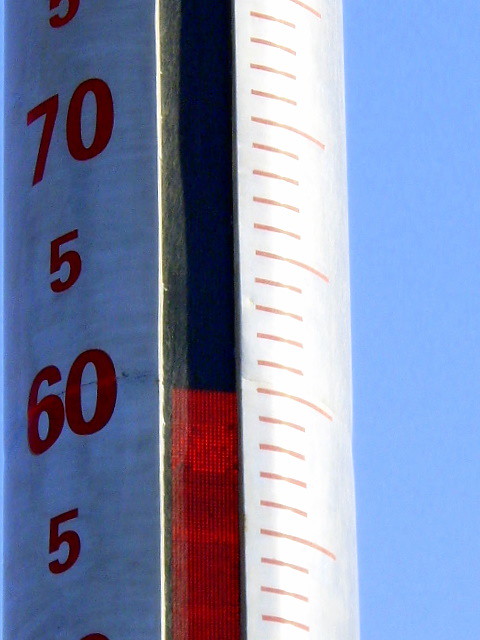The image is a vividly colored graphic illustration prominently featuring shades of blue, white, black, and red. It showcases a close-up view of a wall thermometer, with a design that emphasizes its precise and detailed temperature markings. The thermometer's readings, composed in striking red numbers, stand out against a serene blue background, enhancing readability. Within the thermometer's glass tube, red liquid is visibly rising, aligning with the specified temperature markings. Various meticulously drawn lines and numbers extend from the top to the bottom of the thermometer, providing a comprehensive range of temperature measurements. The current temperature reading is distinctly indicated at 60 degrees, highlighted by the conspicuous red liquid and markings.